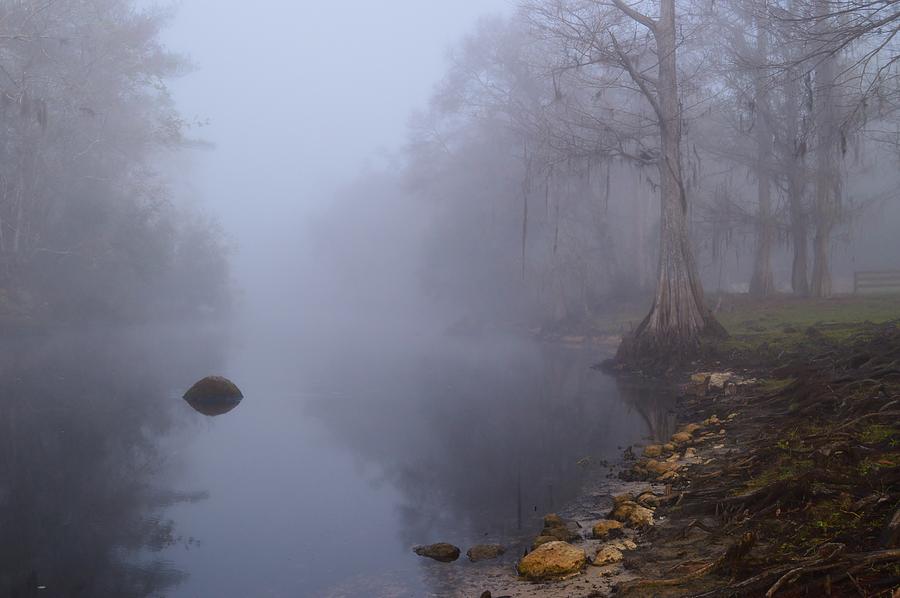This photograph depicts a tranquil, foggy daytime landscape scene featuring a serene body of water, possibly a pond or stream, nestled within a misty forest. The stillness of the water beautifully reflects its surroundings, contributing to the eerie yet calm atmosphere dominated by a grayish tone. On the right side of the image, a rocky shore is lined with large, orange-hued stones, an abundance of roots from nearby trees, and a variety of greenery. Some of these trees appear to be mostly dead with no leaves, enhancing the mysterious ambiance. In contrast, the left side of the water has healthier-looking trees and a solitary, large, hump-backed stone jutting out. The fog becomes thicker in the distance, obscuring the far reaches of the landscape. There's a hint of human presence with what seems to be a bench or a fence barely visible on the extreme right edge, adding a subtle touch of curiosity to the otherwise untouched natural setting.